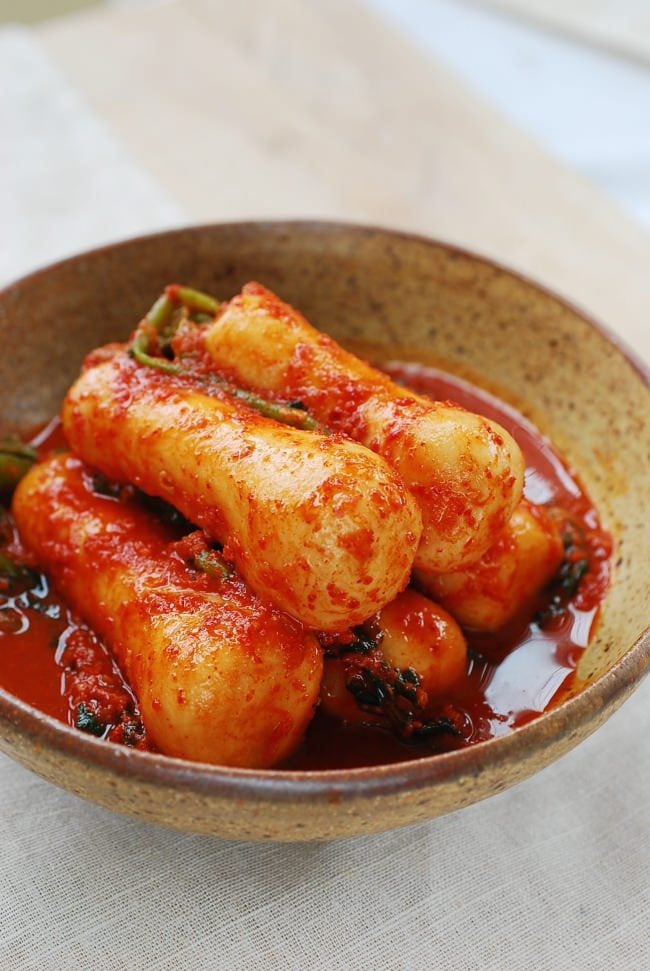The image depicts a small ceramic bowl, tan with brown flecks and a darker brown stripe around the top edge, set on a white linen tablecloth. Inside the bowl, there are precisely formed, tubular white pieces of food which are likely ponytail radishes. These radishes are coated in a vibrant red sauce that accumulates at the bottom of the bowl, creating a glossy shine particularly noticeable on the right side. The dish is garnished with greenery, possibly parsley, with one notable folded leaf positioned toward the top left in the image. The overall presentation of the food and its cultural appearance suggest an unfamiliar, exotic dish.